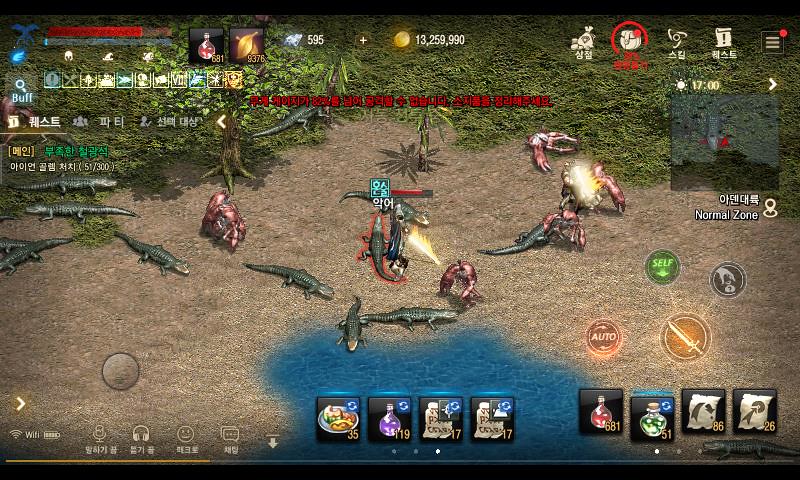This image is a detailed screenshot of a video game, likely a role-playing game with elements of action and strategy. The scene is set in a visually diverse environment with greenery composed of trees and bushes dominating the top part of the screen, transitioning to a sandy and dirt area towards the bottom, highlighted by a central blue water feature. 

In the middle of this vibrant battleground, two or three characters, described as heroes, are engaged in combat, energetically firing their guns at crocodile-like creatures and possibly crabs. This intense action unfolds amidst the lively backdrop of the lush upper area and the tactical lower zone. 

Prominent on the screen are several game interface elements. In the top left corner, there's a blue symbol resembling crossed axes along with a red health bar and a blue bar underneath. Below these, two square icons depict a flask and some golden leaves, while a currency indicator showcases an impressive total of thirteen million, two hundred fifty-nine thousand, nine hundred and ninety (13,259,900). Further, there is a shimmering silver item priced at $5.95. 

The upper center of the screen features Japanese text in red, suggesting additional information or instructions, surrounded by several other icons. On the upper right, more standard game interface icons indicate likely game status such as lives or other resources. 

At the bottom of the screen, a grid of squares implies an inventory system that the character currently has access to, accompanied by icons like a headphone and a smiley face, hinting at communication options like chat. There are also elements suggesting a video recording feature.

Combining the detailed vegetative scenery, the sandy battleground with its aquatic feature, and the busy game interface, this image richly depicts a highly interactive and dynamic video game scene.